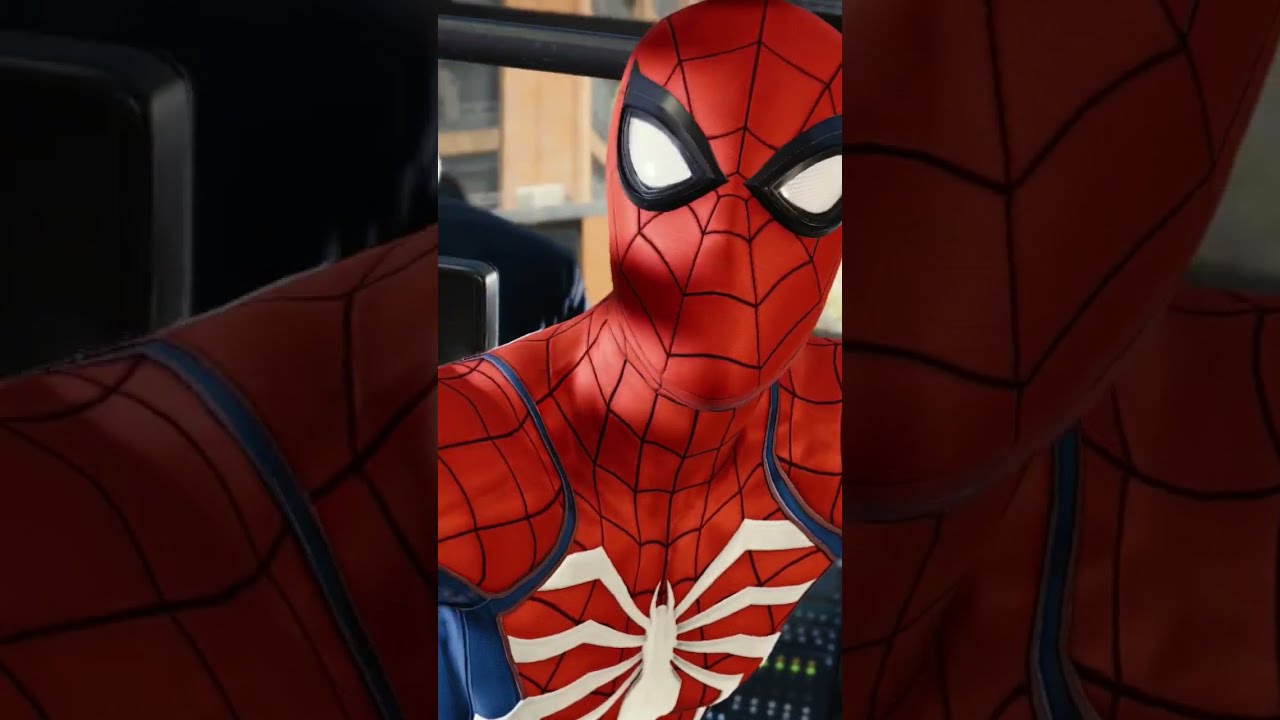The image prominently features a hyper-realistic CGI depiction of Spider-Man, with a strong focus on his face. The central portion of the image is clear and brightly lit, whereas the surrounding area employs a blurry filter that transitions into the sharp center. Measuring roughly 7 to 8 inches wide and 5 inches tall, the composition emphasizes Spider-Man's iconic look. He is dressed in his classic red and blue suit, detailed with intricate webbing patterns. A distinctive white spider emblem adorns the middle of his chest, complete with its thorax and eight legs. His mask showcases the signature large white eyes outlined in black. Spider-Man's arms are slightly out to the side with his shoulders raised, suggesting a poised and alert stance. The background features a building and some equipment, but no text distracts from the main visual. This high-quality image appears almost cinematic, reminiscent of scenes from movies or television programs, and captures Spider-Man looking directly at the viewer.